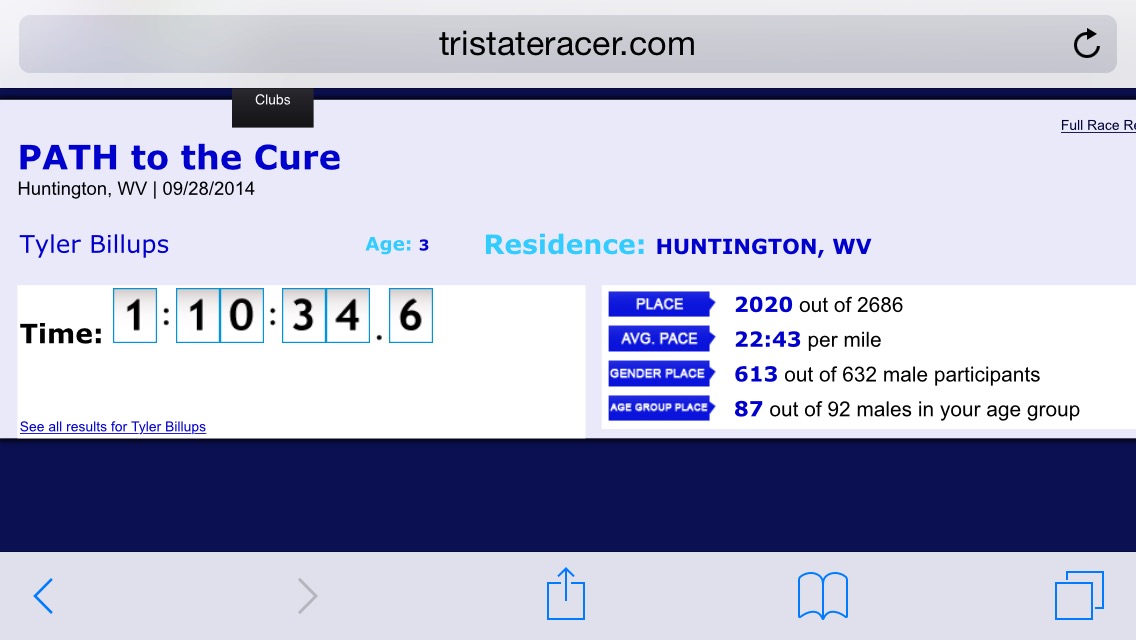The image is a detailed screenshot of a webpage or phone app, titled "tristateracer.com" at the very top in a grey band. Beneath that is a black navigation bar with a "Clubs" button in white text. Following this, there is a dark blue band with the title "Path to the Cure," which includes details such as "Huntington, West Virginia, 09-28-2014" in smaller text.

Centered below this is the name "Tyler Billups" in blue font, indicating an age of 3 years and residence in Huntington, West Virginia. Further down, in black text, it displays a race completion time of "1 hour, 10 minutes, 34.6 seconds." To the right, several blue placards provide additional race statistics: a placement of "2020 out of 2686," an average pace of "22:43 per mile," a gender place of "613 out of 632 male participants," and an age group place of "87 out of 92 males in the age group."

The bottom of the screen features navigation buttons for further interaction with the website or app.